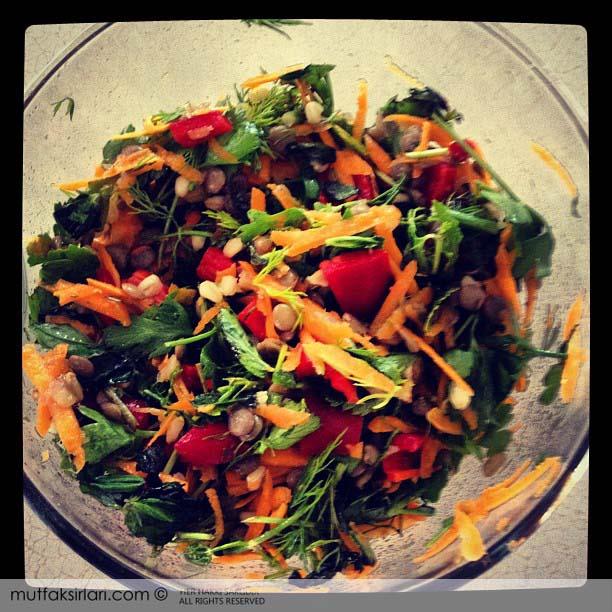This close-up photograph showcases a vibrant salad in a clear glass bowl, resting on a textured tan table. The salad combines finely shredded vegetables with vivid colors and diverse textures. Predominantly, green leaves, which may include spinach, spring mix, or broccolini, form the base. Shredded carrots add a striking orange, while the red hues come from bell pepper wedges and tomatoes. Yellow strips, likely peppers, offer a pop of color, and there are hints of white beans or pine nuts and possibly black olives or seeds mixed in. The bowl features a gray and white pattern with a green accent around its edges. The photograph, outlined in black, carries the website watermark "mutfaksirlan.com" in the bottom left-hand corner. Despite the slightly blurry quality, the image effectively captures the salad's freshness and diverse components.